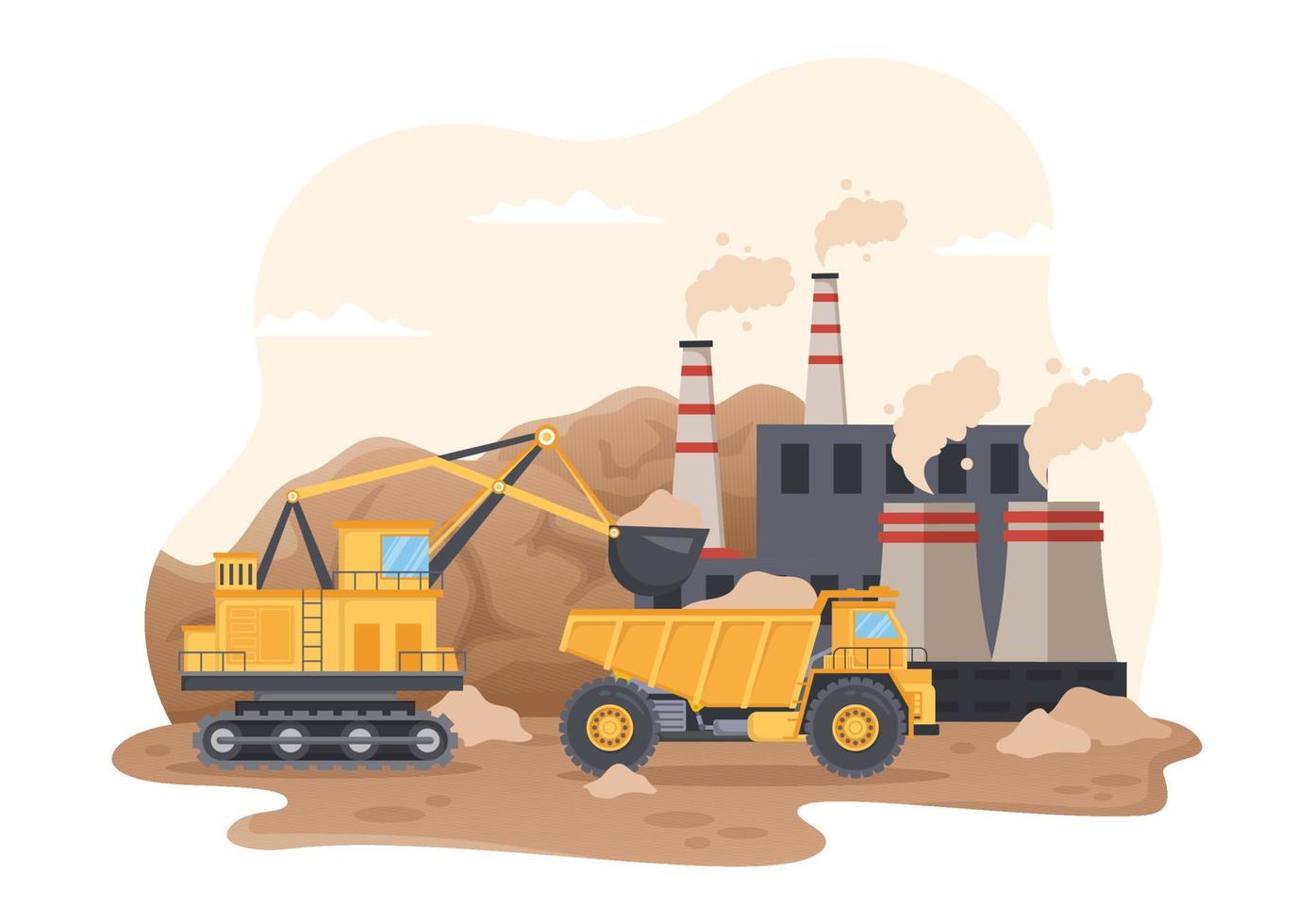This is a detailed graphic of an animated construction site. The scene features a yellow dump truck with large black wheels and yellow rims, loaded with light tan dirt. Positioned behind the dump truck is a yellow backhoe loader with tank tracks and a gray bucket, actively pouring more dirt into the truck. The background showcases several large brown piles of dirt or sand, emphasizing the construction activity.

Dominating the rear of the scene is an industrial plant. The structure consists of a gray building with dark gray windows, and is equipped with multiple cylindrical smokestacks emitting brown smoke. These smokestacks are white with distinct red stripes.

The entire setting is depicted against a light tan sky accented by floating white clouds, one on the left, upper middle, and upper right. The ground features a curved line, suggesting terrain, which separates the construction vehicles and dirt from the sky. Overall, the graphic is characterized by a predominant use of browns and yellows, and lacks any textual elements or borders.